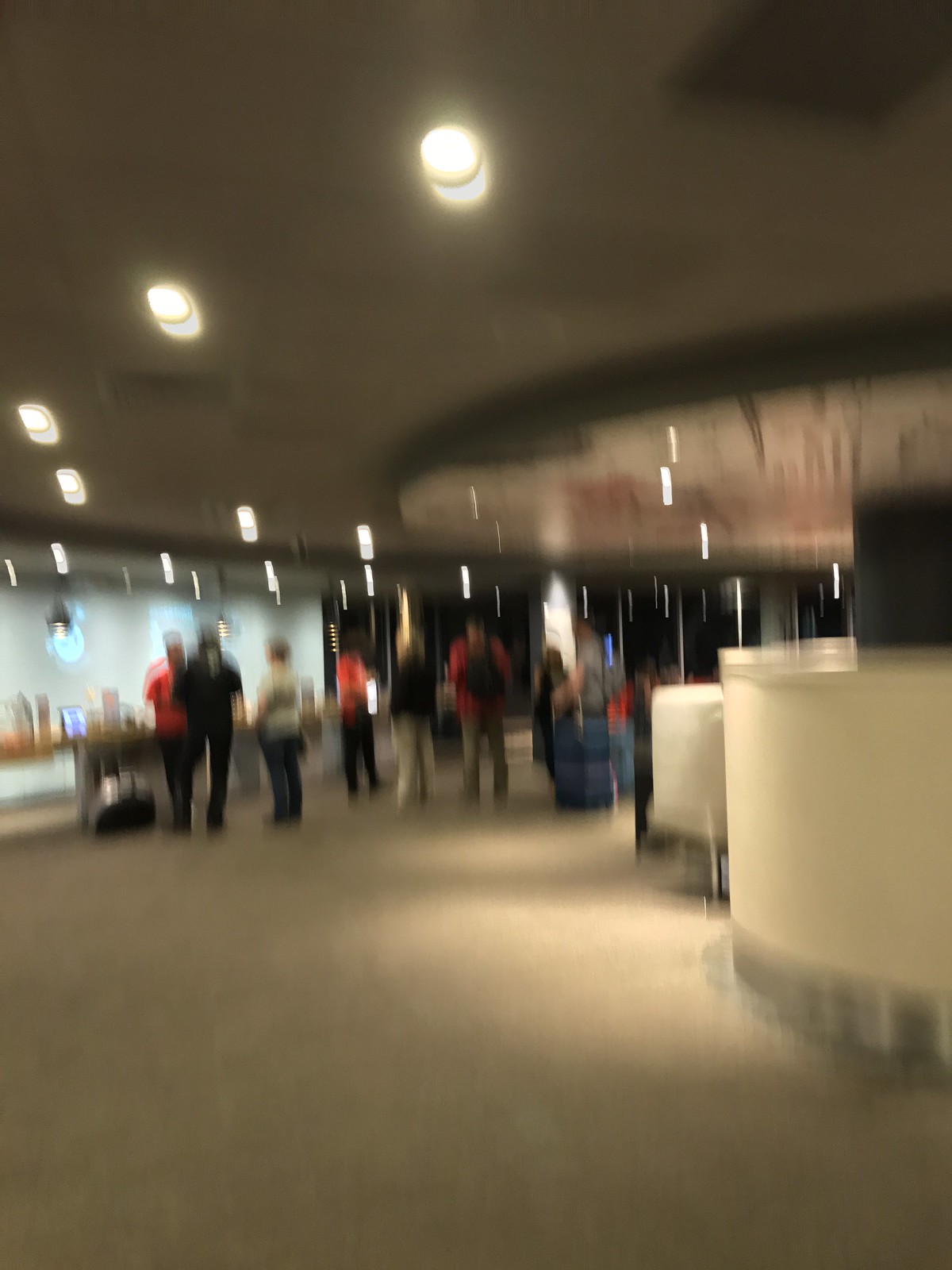This color photograph, though slightly blurry and out of focus, captures an interior view that appears to be an airport terminal. On the left side of the image, several individuals are standing by a rail, some with luggage, including a visible carry-on bag. Across from them, to the right, are cylindrical white booths that likely serve as public customer service stations, although no agents or personnel are visible. The ceiling above features regularly spaced spotlights illuminating the scene below. In the far distance, a structure resembling a gate is faintly discernible, reinforcing the airport setting.